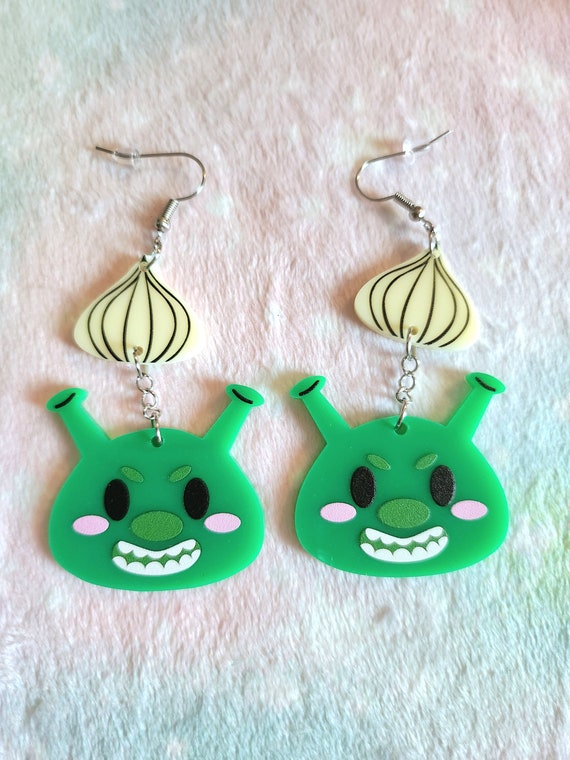This photograph showcases a pair of Shrek-themed earrings, which are displayed on a textured, pink-to-green gradient background that resembles a piece of paper. The background shifts from a pinkish hue at the top to a greenish color at the bottom. The earrings, laid out side by side, rest on a white, fluffy fabric that gives off a fur-like appearance.

Each earring features a green face reminiscent of Shrek, the iconic green ogre. The cartoonish faces smile mischievously, displaying white teeth and blushed pink cheeks. The eyes are entirely black, and an oval nose sits between them. Uniquely, the long, tubular ears—which double as horns—are situated atop their heads, each adorned with a black line.

Attached to the top of the green face via a small silver chain is a charm resembling an onion, complete with lines to suggest texture. Finally, the chain connects to a small metal hook designed to secure the earring in the wearer’s ear. The details and slightly raised features of the face suggest that these earrings are likely handmade, crafted meticulously to capture the whimsical essence of Shrek.